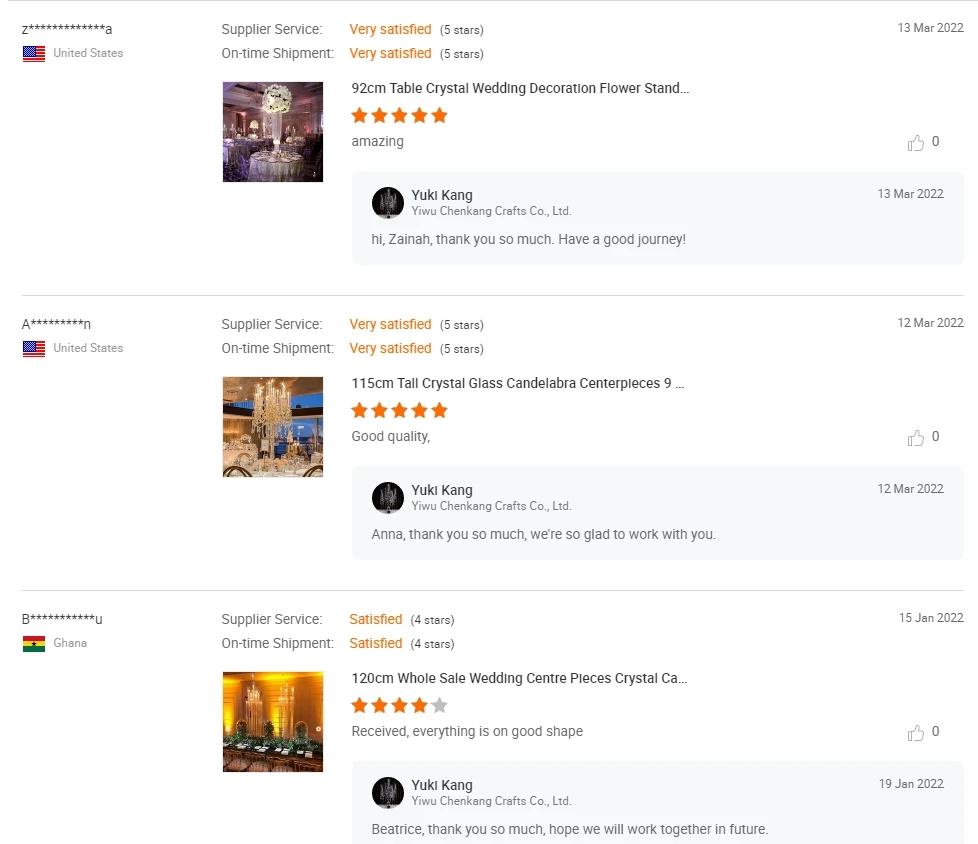In the image, there are three product reviews displayed, each including details on supplier service and on-time shipment. 

1. **Product: 92 cm Table Crystal Wedding Decoration Flower Stand**
   - **Review Date:** March 13, 2022
   - **Ratings:** Both supplier service and on-time shipment categories are rated as very satisfied, with a perfect 5 out of 5 stars, highlighted in orange.
   - **Reviewer:** Yuki King
   - **Comment:** "Hi Zania, thank you so much. Have a good journey."
   
2. **Product: 115 cm Tall Crystal Glass Candelabra Centerpiece**
   - **Review Date:** March 12, 2022
   - **Ratings:** Both supplier service and on-time shipment categories are again very satisfied, with a perfect 5 out of 5 stars.
   - **Reviewer:** Yuki King
   - **Comment:** "Anna, thank you so much. We're glad to work with you."

3. **Product: 120 cm Wholesale Wedding Centerpieces Crystal**
   - **Review Date:** January 15, 2022
   - **Ratings:** Both supplier service and on-time shipment categories are satisfied, with a rating of 4 out of 5 stars.
   - **Reviewer:** Yuki King
   - **Comment:** "Beatrice, thank you so much. Hope we will work together in the future."